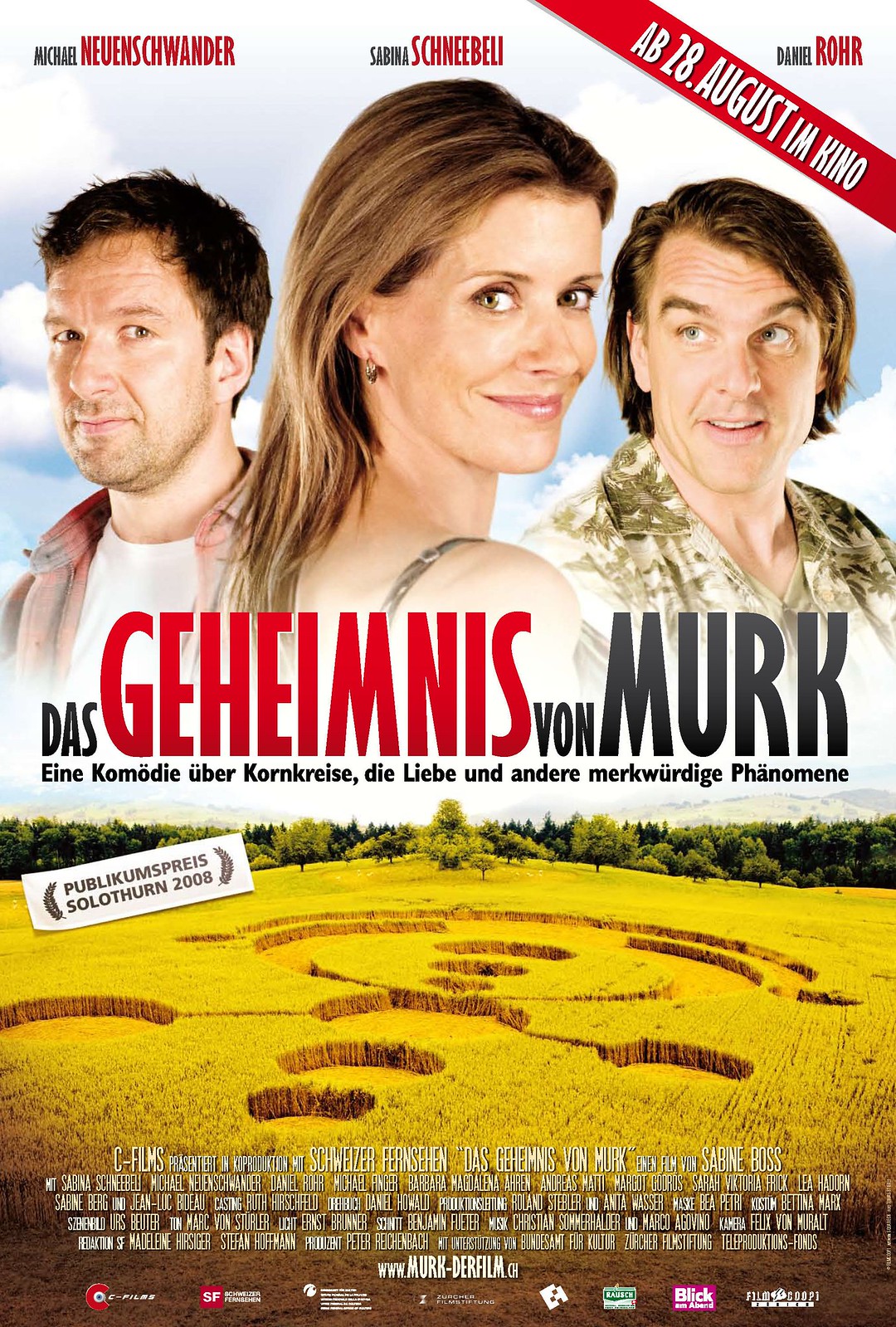The movie poster for "Das Geheimnis von Merck" prominently features three actors at the top against a backdrop of clouds as if they are in the sky. In the center stands a woman named Sabina Schneebelly, with Michael, whose last name appears to be German, on her left and Daniel Rahr on her right. Their names are displayed in lower font, with their first names in black and their last names in larger red font. Michael and Daniel are positioned looking toward Sabina, who is gazing over her shoulder.

The release date of August 28th is shown at an angle across the top of the poster. Below the trio, the title "Das Geheimnis von Merck" is prominently displayed, with the word "Geheimnis" highlighted in bold red letters. The lower half of the poster transitions to an image of a green field marked by intricate crop circles, adding a hint of mystery. Additional information, including movie credits and possible sponsor logos, is listed in white text at the very bottom, alongside a special emblem situated at the top right or left of the field, enhancing the overall design and providing key details about the film.